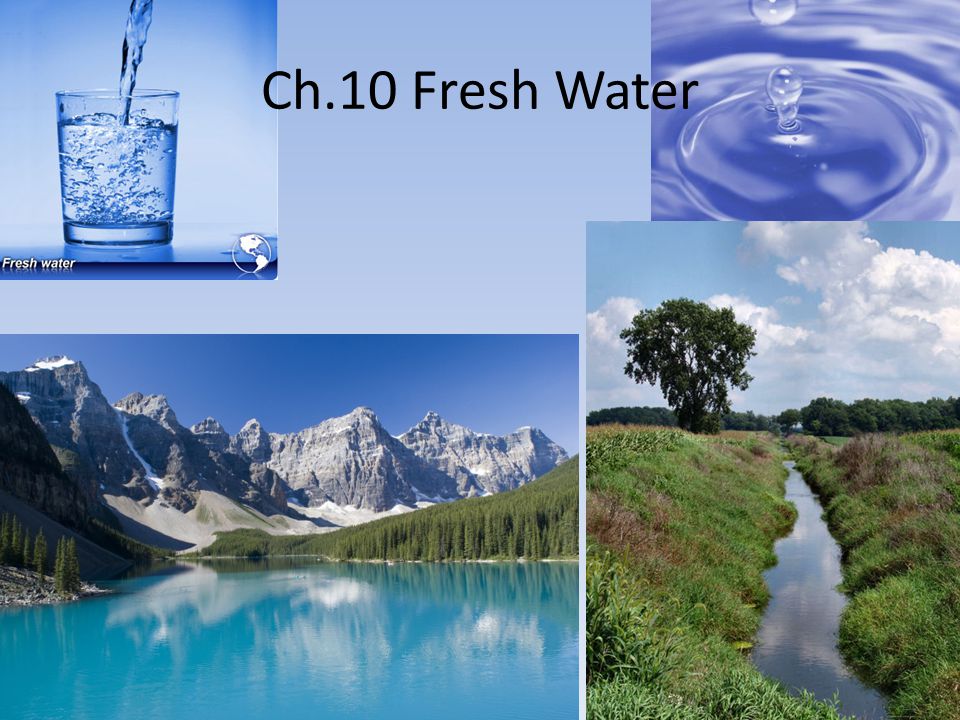This image, titled "Chapter 10: Fresh Water" in black letters at the top center, features a collage of smaller pictures set against a light blue background. In the upper left corner, a clear short glass is being filled with water, partially bubbling up. The liquid appears light blue as it pours into the glass. The upper right corner showcases a serene image of a water droplet creating ripples in a dark blue pool. Stretching across the lower left corner to the middle is a picturesque mountain range with hints of snow, set against a vibrant blue sky. Lush green trees frame the scene, and a strikingly blue lake or creek runs through the foreground. Finally, the lower right corner depicts a peaceful landscape with a tall green tree, green grass, and a small canal under a partly cloudy sky with white, puffy clouds.